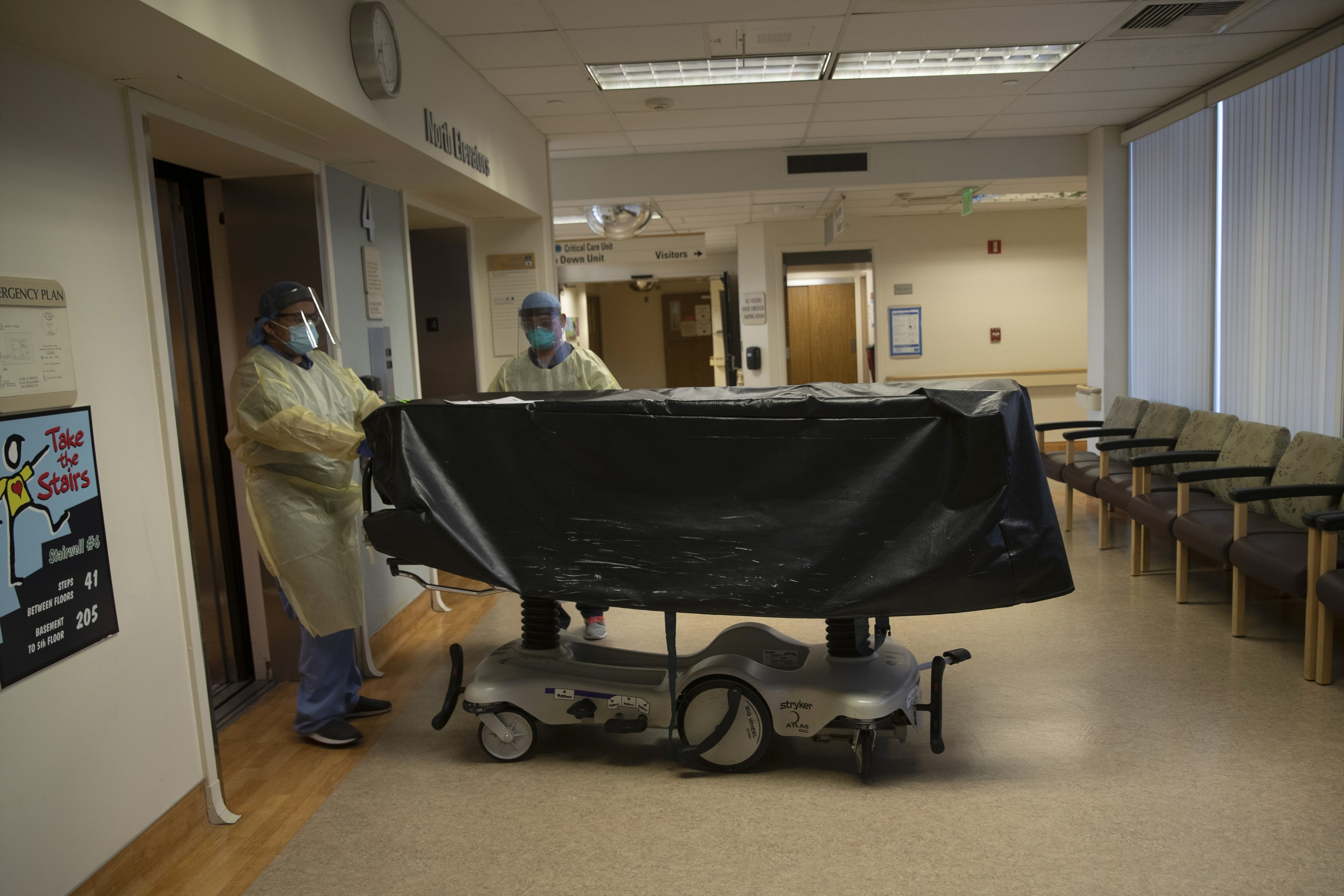In this detailed indoor hospital scene, two medical personnel are the central focus, dressed head-to-toe in protective gear which includes scrubs overlaid with translucent yellow disposable gowns, face masks, and clear face shields. They are seen maneuvering a large, metallic gurney covered with a heavy black tarp, suggesting the possibility of transporting a deceased patient. The hospital setting is unmistakable with its cream-colored walls and an array of signage, including a prominent sign urging the use of stairs and another marking an elevator as number four, which reads "north something" above it. There is a visible clock on the left wall. To the right, a hospital hallway extends back towards other areas populated with chairs and windows, the latter adorned with closed blinds. The duo appears to be guiding the gurney into an elevator, captured in the midst of their critical medical duties.